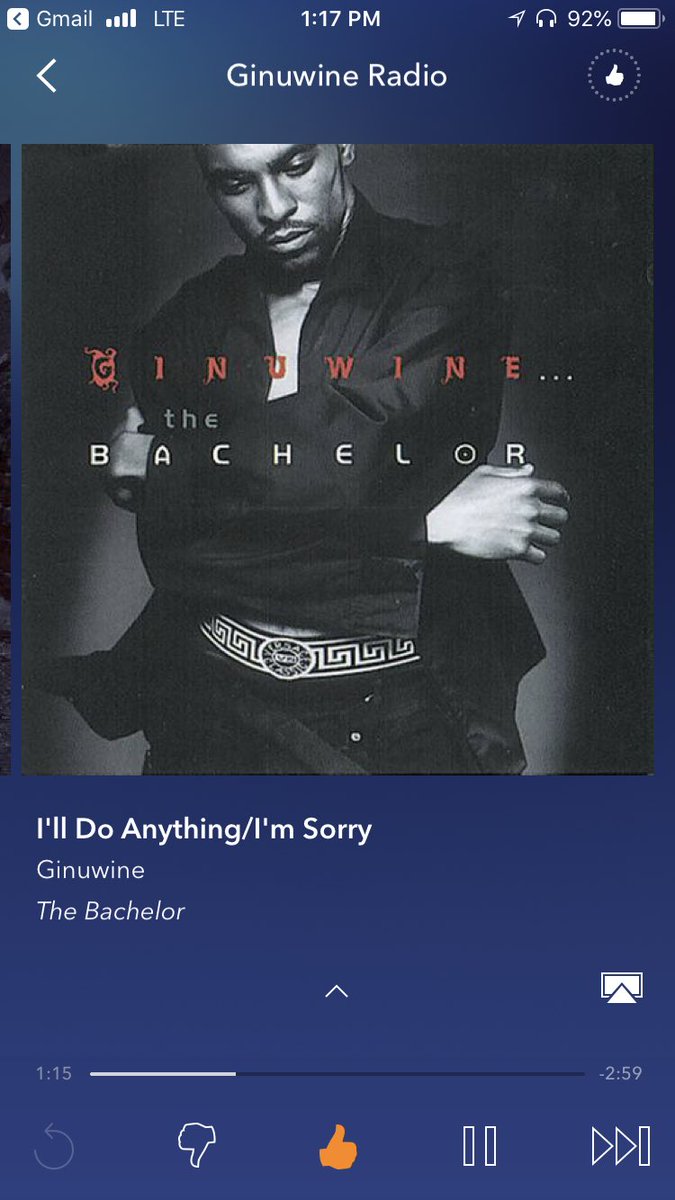The image appears to be the cover art for an album by a black male artist named Genuine. The top section prominently features the text "Genuine Radio" twice, indicating perhaps a radio station or a music service. The upper right corner shows the time at 1:17 PM and a battery life of 92%. The phone network is running on LTE, and there is a back arrow icon at the top, suggesting this is being viewed on a smartphone.

The album cover shows Genuine, dressed sharply in a black suit with a black and white wide belt, standing with his arms folded and wearing a serious expression while looking down. His name, "Genuine," is highlighted in red text, while the album title, "The Bachelor," is printed in white. The background of the image transitions from blue at the top to blue at the bottom.

Beneath this, the songs "I'll Do Anything/I'm Sorry" are listed, indicating they are part of the album. A progress bar shows that the song has been playing for 1 minute and 15 seconds out of a total length of 2 minutes and 59 seconds. An orange thumbs-up icon is visible, likely indicating a positive rating for the song.

An additional white thumbs-up icon within a circle is present, adding another element of interaction or approval.